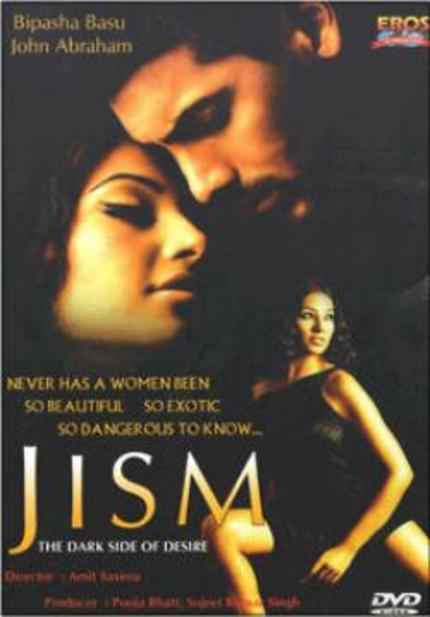This is a DVD cover for the movie "JISM: The Dark Side of Desire." The background is dark, featuring a romantic close-up of a man and woman, their faces nuzzled together and eyes closed, suggesting an intense, intimate connection. Below them, another woman, dressed in a short, off-the-shoulder black satin dress, strikes a dynamic, dance-like pose, one leg extended as if in a lunge. The title "JISM" is prominently displayed, followed by the subtitle, "The Dark Side of Desire." A tagline on the cover reads, "Never has a woman been so beautiful, so exotic, so dangerous to know." The top of the cover features the names of the lead actors, Bipasha Basu and John Abraham. Additional details include a blurry DVD logo at the bottom right and an Eros logo at the upper right. The cover's quality appears to be compromised, suggesting it may be a reproduction or copy.